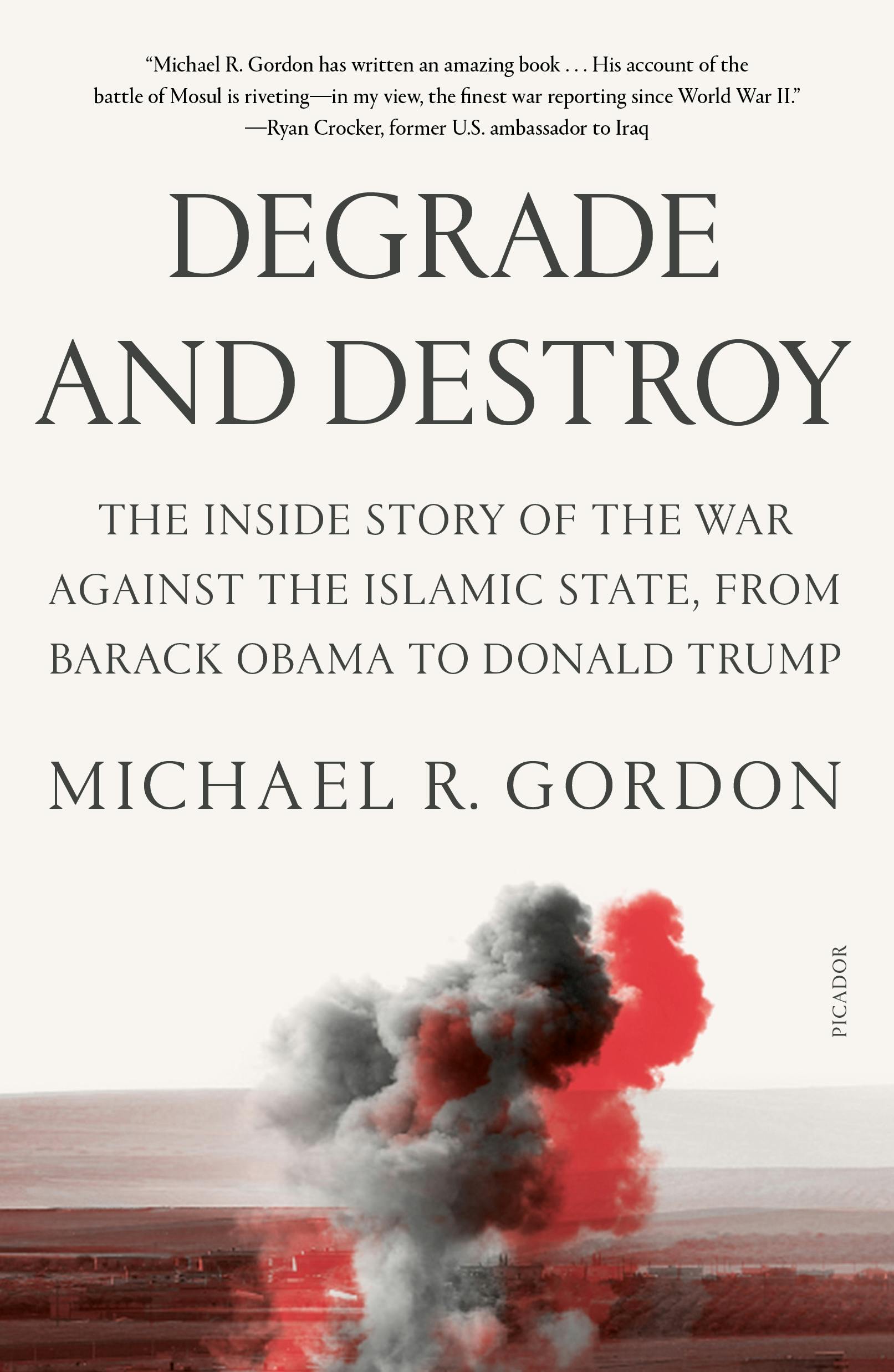This photograph depicts the cover of the book "Degrade and Destroy: The Inside Story of the War Against the Islamic State from Barack Obama to Donald Trump" by Michael R. Gordon. The cover is primarily an eggshell or cream color, with the bottom section featuring a striking, rusted blood-red hue. At the top of the cover, there is a review from Ryan Crocker, former U.S. Ambassador to Iraq, which states, "Michael R. Gordon has written an amazing book. His account of the Battle of Mosul is riveting. In my view, the finest war reporting since World War II." Beneath this endorsement, the book's title is displayed in large print, followed by a subtitle in smaller font. Michael R. Gordon’s name appears prominently below the title. At the bottom of the cover, there are two plumes of smoke; one is a solid gray, and the other matches the rusted blood-red background, creating an opaque silhouette. The scene suggested by the smoke plumes evokes a sense of desolation, likely over a desert landscape, under daylight.